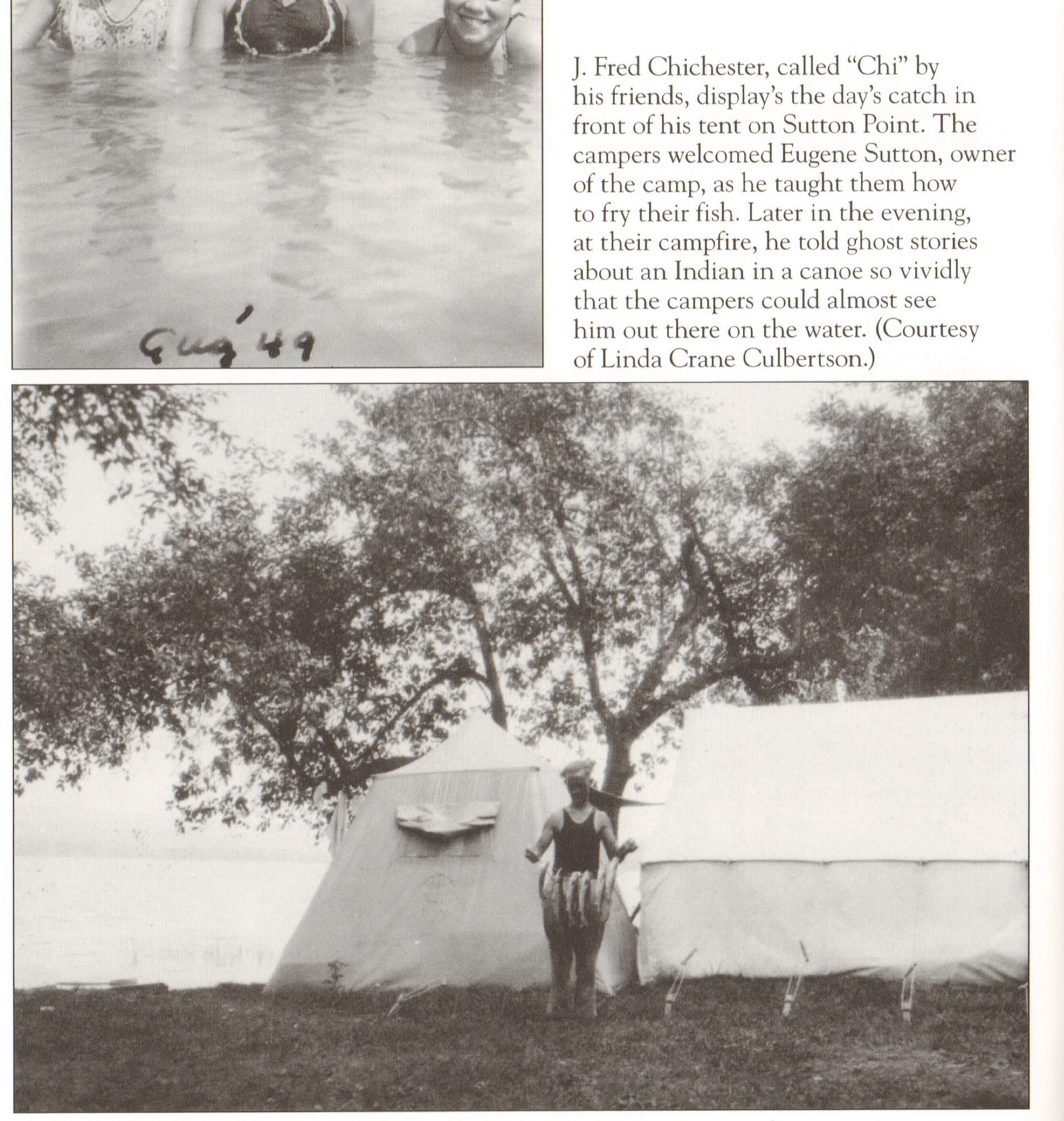The image features multiple photographs and a detailed caption in black text at the top right. The first photograph, situated at the top left, shows three individuals chest-deep in water, with "G.U.G. '49" marked in black marker, indicating the date as August of 1949. The caption reads: "J. Fred Chichester, called Chee by his friends, displays the day's catch in front of his tent on Sutton Point. The campers welcomed Eugene Sutton, owner of the camp, as he taught them how to fry their fish. Later in the evening, at their campfire, he told ghost stories about an Indian in a canoe so vividly the campers could almost see him out there on the water, courtesy of Linda Crane Culbertson." The bottom half of the image showcases J. Fred Chichester holding a string with multiple fish strung through it. He is dressed in long pants, a sleeveless tank top, and a hat, standing in front of two tents with a tree behind them, near a lake.